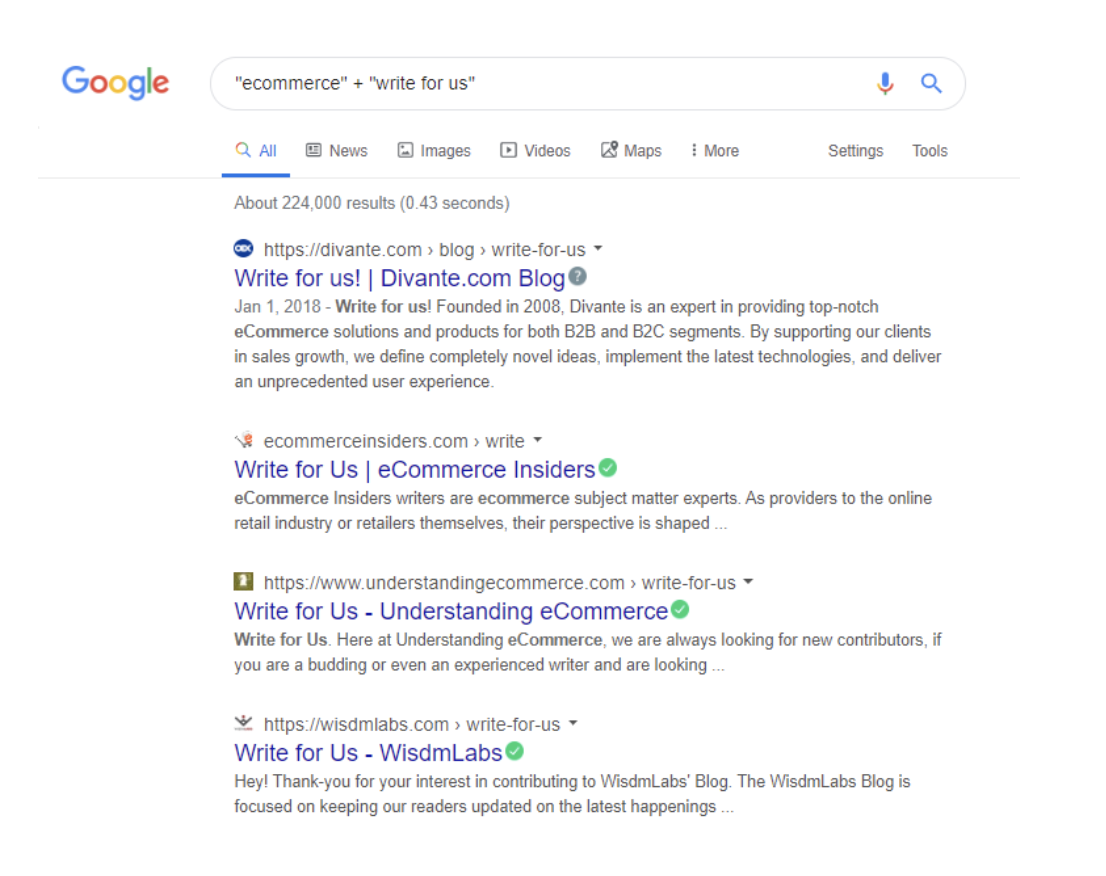This screenshot captures a Google search page interface. In the upper left-hand corner, the distinctive Google logo is prominently displayed, featuring its iconic rainbow-colored letters in blue, red, yellow, and green. Adjacent to this, on the right-hand side, is the search box that includes both a microphone icon and a magnifying glass icon, signifying voice and text search options respectively. The search query entered in the box is "e-commerce" in quotes followed by "write for us" in quotes.

Below the search box, a horizontal menu lists various categories, each accompanied by a small icon. From left to right, these categories are: All (house icon), News (newspaper icon), Images (camera icon), Videos (play button icon), Maps (map pin icon), followed by a vertical line separator, then More. Further right are options labeled Settings and Tools.

Directly underneath, the search results summary indicates approximately 224,000 results found in 0.43 seconds. The results section features a series of four entries. Each result lists the website above the title, with the title in blue. The first search result reads "Write for us - Devante.com Blog," accompanied by a brief description. The second result, titled "Write for us - Ecommerce Insiders," is marked with a green circle containing a white checkmark, denoting its credibility. The third result shows "Write for us - Understanding Ecommerce," also noted with the green verification circle. Finally, the fourth result, "Write for us - WISDM Labs," includes a matching green verification icon, ensuring its authenticity as well. Each result provides further context about writing opportunities in the e-commerce niche.